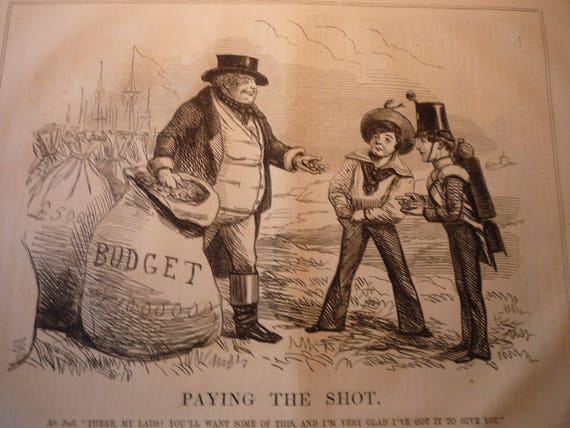The image is a detailed vintage political cartoon, likely from the early 1900s or 1920s, illustrated in sepia tones. The scene features a large, portly gentleman wearing a black top hat, a black suit, a faded or white waistcoat, black and silver boots, and a black and gray scarf. He stands prominently in the foreground, leaning his right hand into a massive sack labeled "BUDGET" with "100,000 pounds" written underneath. In his left hand, he holds out several coins.

To the right of the gentleman are two young boys standing on grass. One boy is dressed in a sailor's uniform, complete with a hat, shirt, and cravat, and is seen reaching into his pocket, possibly to find coins. The other boy is clad in an old-style military uniform with a rucksack and bedroll, having already produced some coins.

In the background, birds can be seen flying, and to the left, a ship with steam billowing from it is visible. The sacks next to the gentleman are marked with "50,000 pounds," and all are tied up neatly.

At the bottom of the drawing, in capital letters, the text reads "PAYING THE SHOT," followed by a dialogue: "MR. BULL, THERE MY LAD, YOU'LL WANT SOME OF THIS, AND I AM VERY GLAD I'VE GOT IT TO GIVE YOU." The entire piece is rendered in black pencil, giving it a classic, textured appearance typical of the era's newspaper comics.